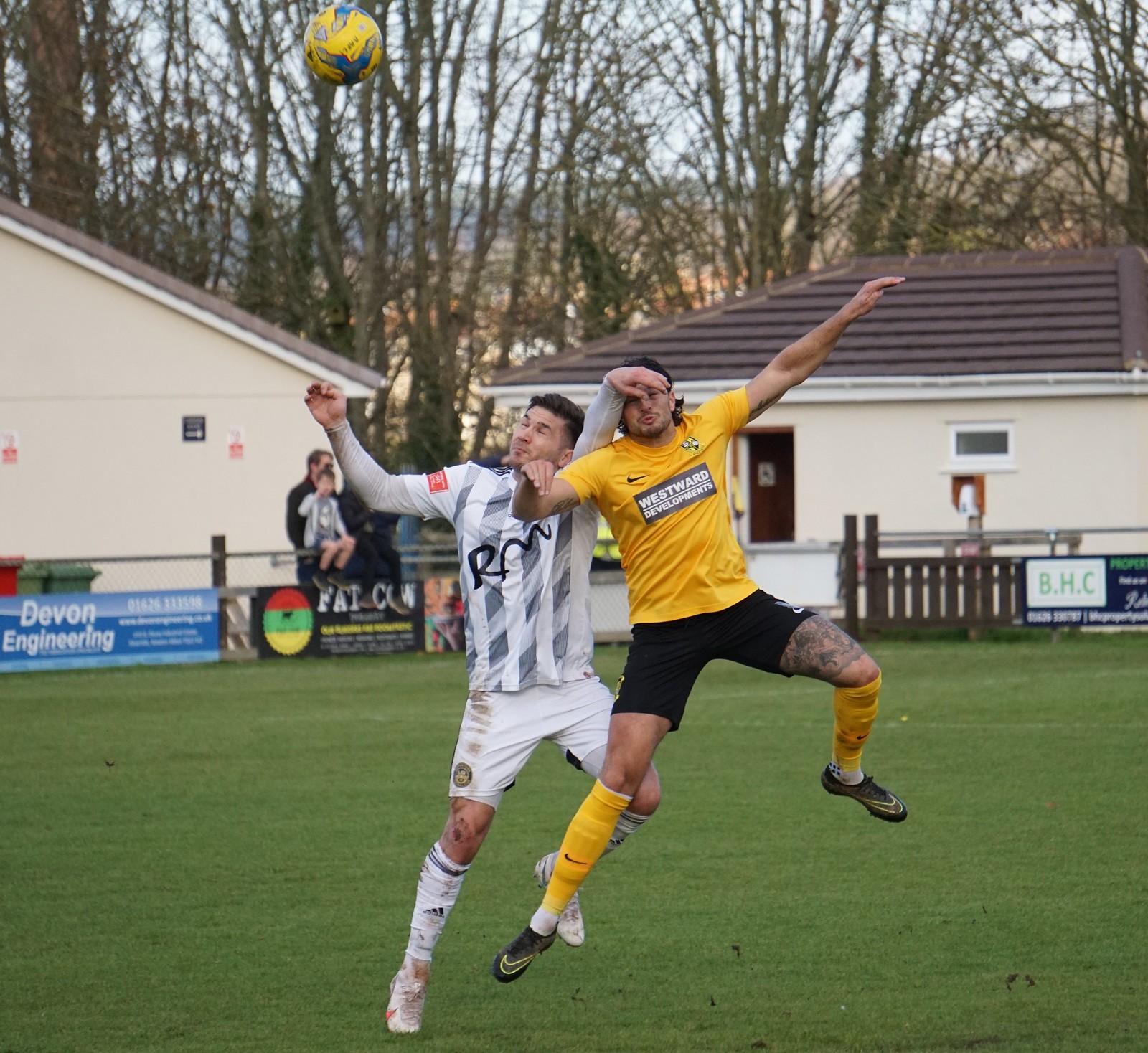In the vibrant color photograph, two soccer players compete fiercely for a high soccer ball positioned in the upper left-hand corner of the image. The player on the left, dressed in a white and silver uniform, reaches up with his right hand while using his left hand to shield the forehead of the opponent beside him. The opponent, clad in a black, gold, and white uniform, is captured leaping into the air amid their intense struggle.

The action unfolds on a lush green grass pitch, with a backdrop that adds context to the scene. Two white buildings with brown roofs stand prominently in the background, possibly serving as restrooms. Fences and blurry onlookers frame the scene, adding to the atmosphere. Numerous advertisement signs pepper the background, although they are hard to read clearly. Notably, a blue and white sign for Devon Engineering and a multi-colored one for Fat Cow catch the eye. Additionally, a white sign for BHC is visible on the right, albeit partially blurred. The setting is completed by visible patches of sky and a scattering of trees in the right-hand portion of the background, providing a peek into the surrounding environment.